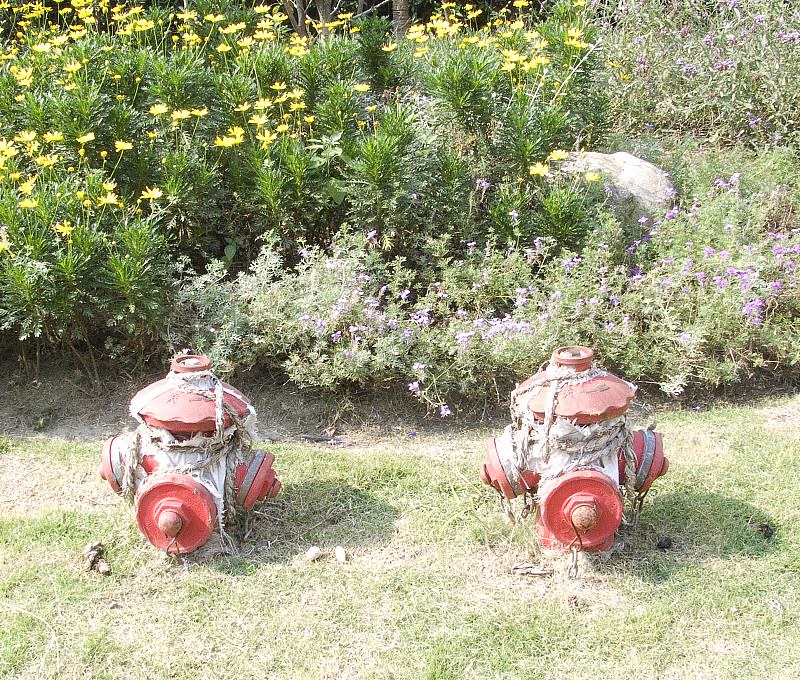This photograph, likely taken outdoors on a sunny day, features two short red fire hydrants set in a grassy field with occasional light brown patches. The fire hydrants are old and deteriorating, ensnared in thick, deteriorated white rope or plastic wrap, suggesting they might no longer be in use and could be ornamental. Scattered around them are small brown stones and what appears to be dog feces. The backdrop of the image is a lush garden composed of various bushes and shrubs, adorned with wildflowers. The bushes are vibrant, some with bright green leaves and clusters of tiny yellow flowers, while others have less vivid leaves and soft pink or light purple flowers. The high contrast and possible overexposure give the photograph a slightly washed-out appearance, blurring fine details and lending a dreamy quality to the floral display. Near the right side, a sizeable gray rock rests amongst the bushes. This scene may represent the back end of a yard or a park where these fire hydrants serve as quirky garden fixtures amidst the lively plant life.